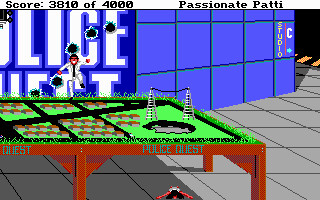The image is a screenshot from a vintage video game that exudes a nostalgic, retro charm. The scene depicts a room with a gray-tiled floor and walls clad in blue tiles, reminiscent of a classic 8-bit or 16-bit era. A brown and green table occupies the foreground. The green surface of the table appears to house a miniature town or perhaps a detailed train set, inviting the player's imagination to delve into the intricate diorama.

Above the scene, white text displays, though it is partially obscured, rendering the full message indecipherable. Another intriguing detail is the presence of what seem to be bullet holes punctuating the white lettering on the wall, adding an element of mystery or past conflict.

Dominating the upper portion of the screen, the player's score of 3810 out of a possible 4000 is prominently displayed, alongside the phrase "Passionate Paddy," which could be an intriguing nickname or title associated with the player's character or status within the game.